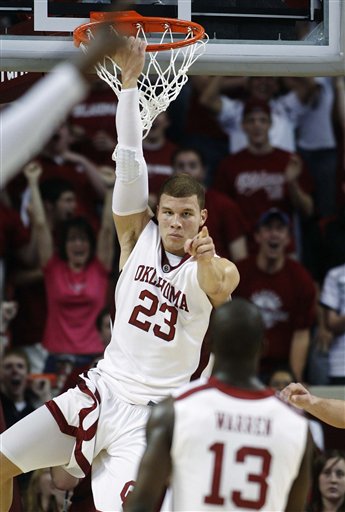This tall, rectangular photograph captures a dynamic moment in a basketball game featuring an Oklahoma player, number 23, who has short brown hair and light skin. He is hanging onto an orange basketball hoop with a white net, his right arm gripping the rim while his left arm points directly forward, possibly at an opposing player. Number 23 wears a distinctive white and red uniform, complete with a white sleeve on one arm. The hoop, slightly left of center at the top of the image, is attached to a black backboard with a gray border. Standing in front of him in the bottom right corner is another Oklahoma player, number 13, who has black skin, no hair, and a similarly colored jersey displaying the name "Warren." The image is set against a lively background of a cheering crowd, with particular emphasis on an enthusiastic woman in a red shirt with her arms raised. This scene likely captures an intense and celebratory moment, perhaps following a blocked shot or a scoring play.